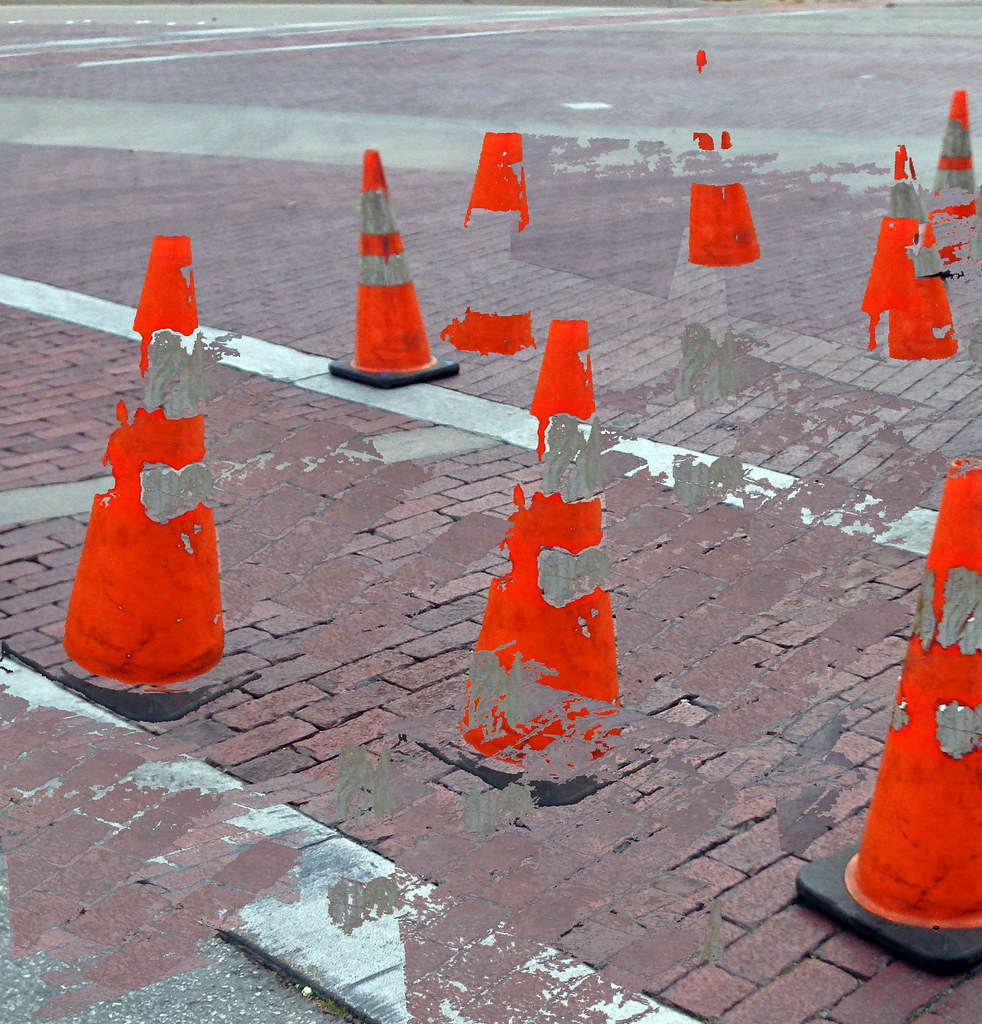This photograph, captured during the daytime in excellent lighting conditions, has been digitally altered to create a surreal scene. It features several orange traffic cones with black bases that are positioned on a brick surface of a mauve-pink hue. Unusually, sections of the cones—particularly some center and bottom portions—are missing, revealing the underlying brick texture instead of the expected orange. In a peculiar twist, this brick coloration appears to bleed onto an adjacent gray concrete area, further enhancing the surreal effect. Adding to the oddity, some of the cones appear to be floating midair. Despite the apparent visual manipulations, the image quality remains crystal clear, making it easy to identify each object despite the poorly executed Photoshop effects.